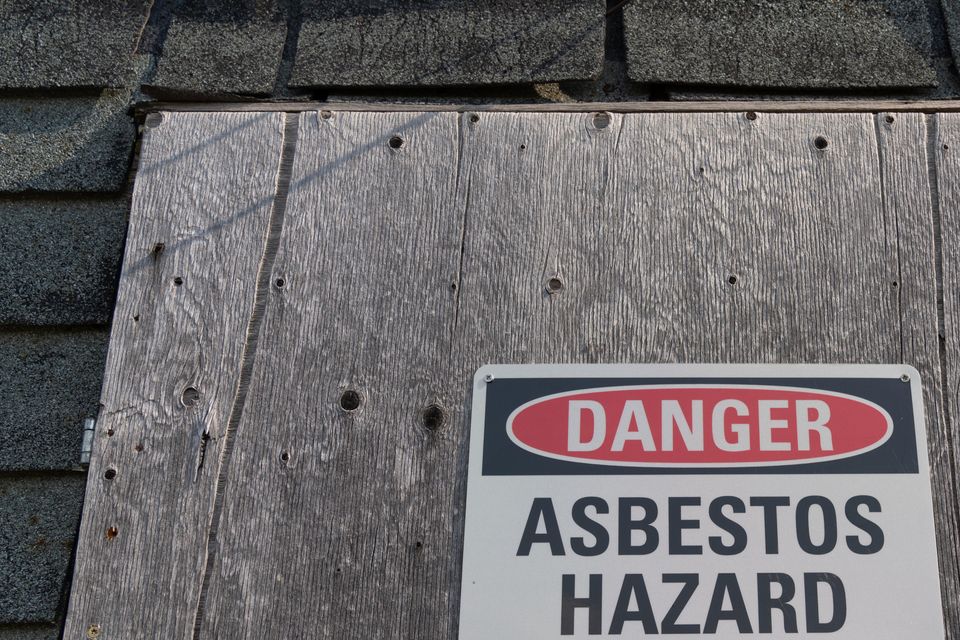A close-up color photograph reveals a section of a weathered building. Dark gray to almost black shingles frame the left side and top of this image, highlighting their rectangular shape. In the center, there's an old piece of plywood, visibly worn and weathered, featuring several knots and a significant crack along the left side. A metal hinge attaches this piece of wood to the shingles, suggesting it might be a small door or panel. Dominating the lower right section of the photograph is a rectangular white sign, adorned with a red oval containing the word "Danger" in white. Below this, the sign reads "Asbestos Hazard" in black text. Shadows cast by the sunlight provide additional texture and depth, emphasizing the predominant shades of gray in the composition.